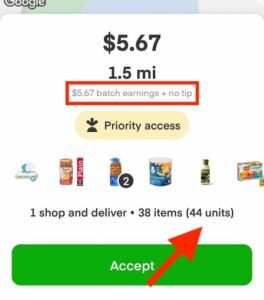The image depicts a detailed interface, possibly from a delivery app. At the very top of the interface, there is a thin bar. On the left side of this bar, the word "Google" is displayed. The bar itself transitions from a greenish hue on the left to a bluish hue that dominates most of the space. On the right side of the bar, the background turns white. Within this white section, there is a double space followed by the text "$5.67." Then, it shows "1.5 MI" separated by a space.

Below this top bar, there is a white rectangle outlined with a red border that reads "$5.67 batch earnings plus no tip." Next to it, there is a yellow rectangle with rounded edges that says "priority access" and includes an icon of a bell with a downward-pointing arrow next to the bell.

The next section displays six different items presumably for delivery. One of these items is marked with a white number "2" within a black circle. This is followed by the text "1 shop and deliver," a black dot, and then "38 items" with "44 units" in parentheses. Highlighted in green is the word "accept," accompanied by a red arrow pointing to the right.